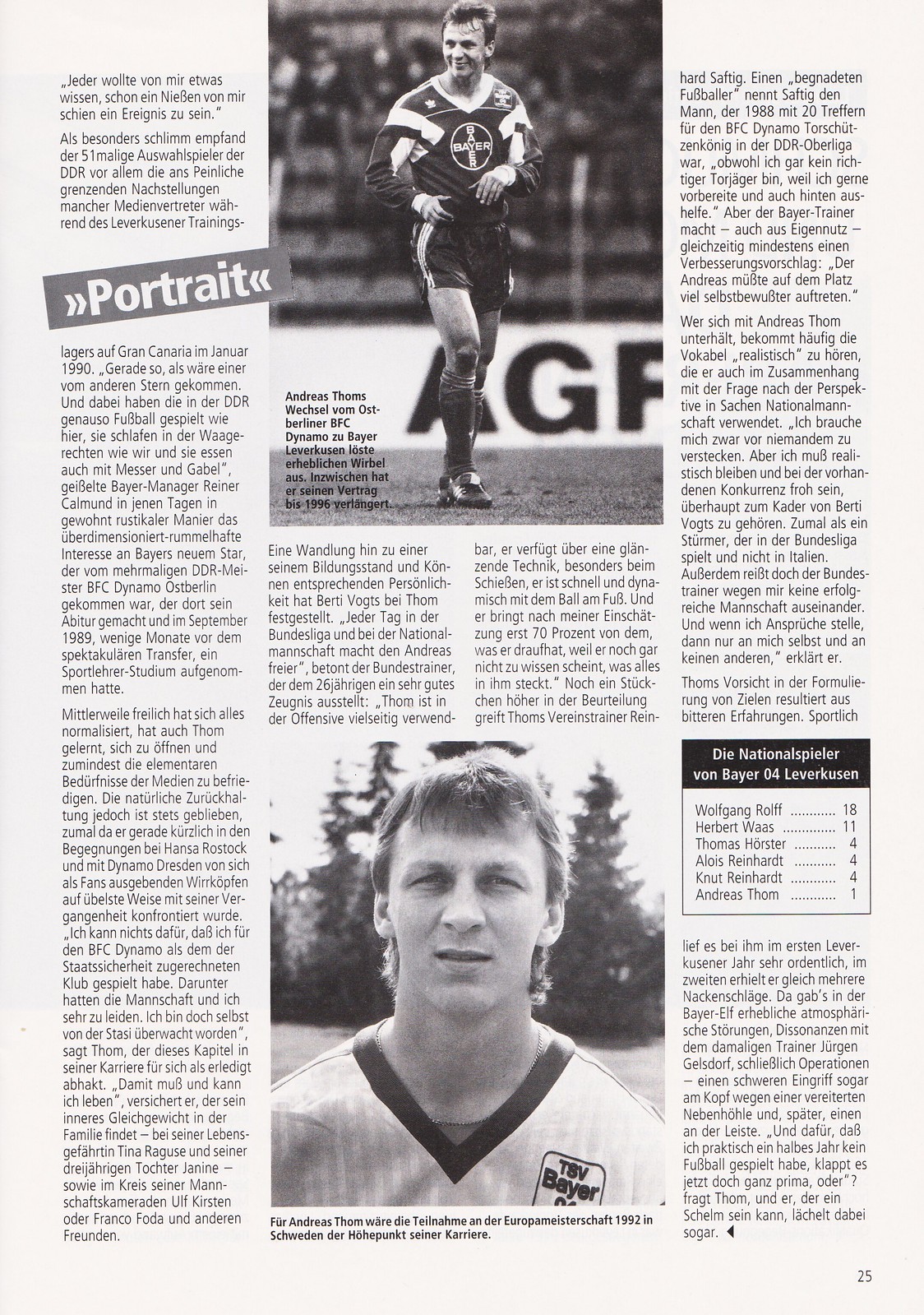The image is a black and white page that appears to be taken from a German newspaper or sports magazine. The page itself is showing its age with an off-white color. The main article, written in German, seems to focus on a soccer player from the TSV Bayer team. At the top of the page, there is a photograph of the soccer player, captured running and smiling on the field. He is wearing a jersey with the name "Bayer" on the front, featuring dark sleeves, black shorts with a white stripe, and is visible against a backdrop of spectator stands and advertising boards displaying the letters "AGF".

Below this, there is another black and white photograph of the same player, but it is more of a headshot, likely positioned for photo identification or a sports card. This second image shows the player squinting slightly at the camera with evergreen trees in the background, resembling a park area. The player is again wearing the TSV Bayer team jersey. To the right of this image is a box containing some statistics related to the player. Additionally, above these pictures, there is a banner at an angle with the word "Portrait" in white print on a gray background, providing a headline for the article.